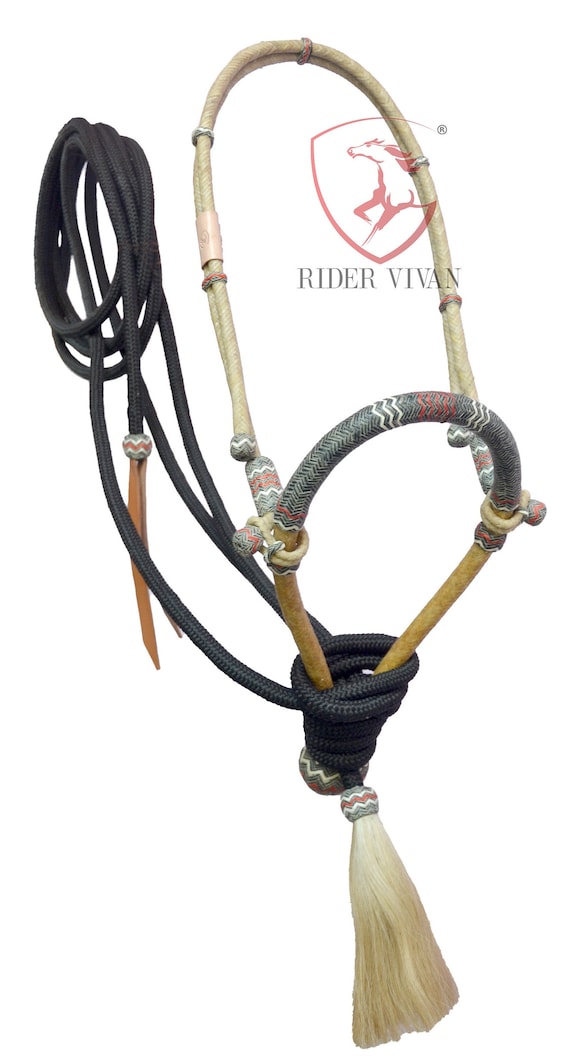The image depicted is a bitless bridle for a horse, prominently featuring a braided cord construction. The bridle, made of a durable and heavy braided cord, fits snugly behind the horse's ears and extends over the muzzle, ultimately being secured in a knot beneath the horse's chin, ending with a decorative tassel. Integral to the bridle are the reins, composed of a black braided cord, that loop underneath the portion covering the muzzle. These reins culminate in a touch of leather fringe and a bead. The background of the image is white, and there is a logo at the top – a red shield containing a drawing of a running horse accompanied by the text "Rider Viben."